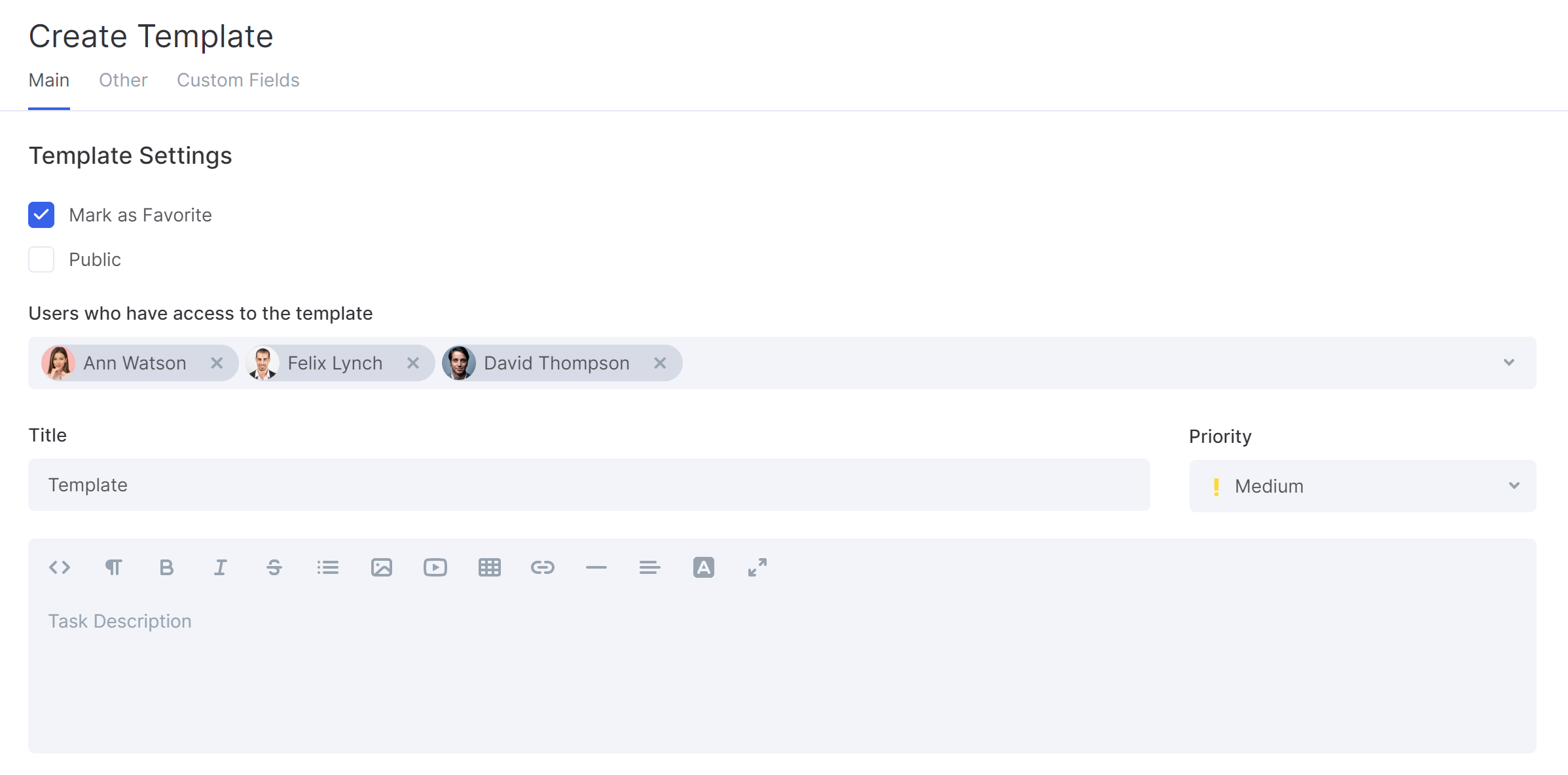This is a digital screenshot of a user interface for creating a template. At the top of the interface, the header reads "Create Template." Below the header, there are several sections and buttons: a main button, an "Other Button," and an area for custom fields. 

Further down, there is a section titled "Template Settings." Within this section is a blue and white checkbox labeled "Mark as favorite," which is checked. Next to this is a "Public" button that is currently unchecked. Beneath these options, a list titled "Users who have access to the template" appears, displaying three users.

The first user listed is Ann Watson, a white female with dark hair who appears to be around 30 years old. Following her is Felix Lynch, a white male who appears to be approximately 40 years old. The last user is David Thompson, a male with dark hair who seems to be about 35 years old.